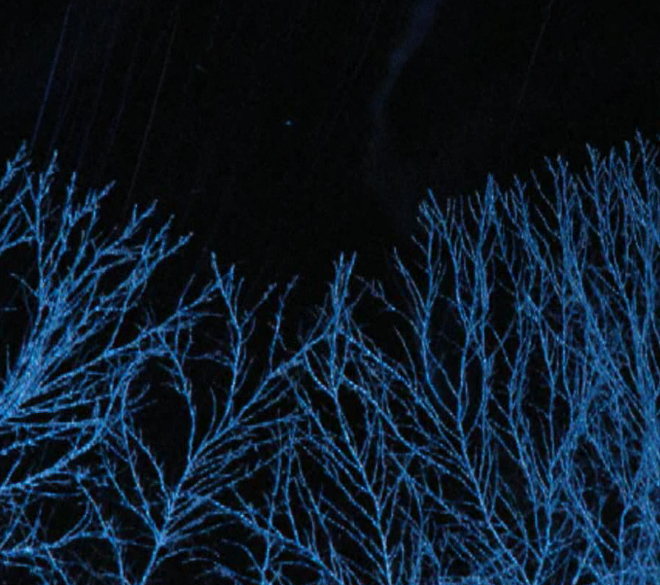The image captures a striking nighttime scene from ground level, gazing upwards at a sky enveloped in darkness. In the foreground, the intricate silhouettes of tall trees dominate, their bare, branch-laden forms starkly set against the inky black sky. These branches, illuminated by a bluish-white light source positioned below, exhibit a complex, web-like structure reminiscent of the nervous system, with multiple offshoots extending from the main limbs. Most of the branches appear stringy and are distributed unevenly across the frame, taller on the right, dipping in the middle, and rising again on the left. The sky is largely void, with a single dim star positioned slightly left of center and near the top, adding an isolated point of light to the somber tableau. Wisps of indistinct, light-toned streaks stretch from the trees into the black expanse, adding further texture to the scene. The overall image conveys a sense of quiet, wintry solitude.